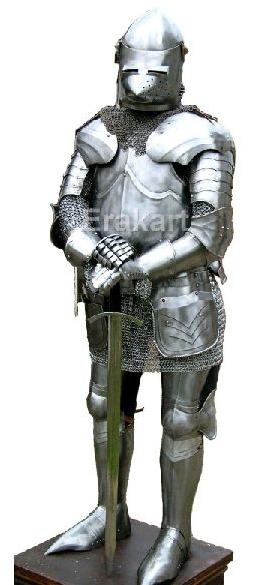This image depicts a meticulously crafted knight's armor standing on a podium. The armor, made of silvery metal and polished to a sheen, covers the suit entirely from head to toe. The helmet features a domed, cone-shaped top with slits for the eyes and small openings for breathing. Chain mail mesh is visible underneath the metal plating, draping over the shoulders, chest, arms, and continuing down to the thighs. Additional metal plates protect the shoulders, arms, fingers, legs, and feet. The knight holds a large sword with both hands, its tip resting on the podium. The podium itself appears to be wooden or possibly black, providing a sturdy base for the display. Positioned just above the hands on the breastplate, there is a watermark that reads "ERAKART," potentially indicating the creator of this piece. The entire setup is presented against a plain white background, suggesting a digital rendering or a museum display, with no additional context to determine the exact size or location.